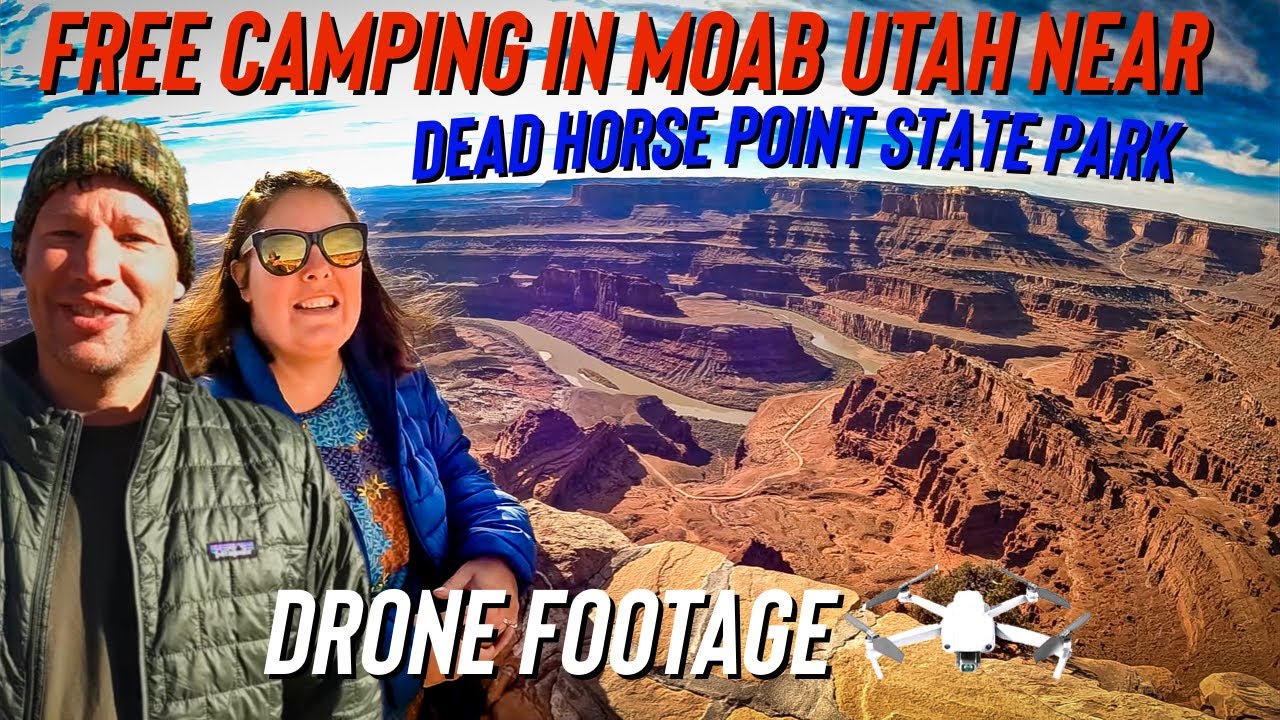This real-life photo advertisement highlights free camping in Moab, Utah, prominently showcased at the top in bold red letters with a black shadow. Directly below, blue letters with a black shadow reveal the inviting proximity to Dead Horse Point State Park. Framing the picturesque scene, an older man and woman stand on a scenic ledge. The man, wearing a camo green beanie and a gray bomber jacket, smiles warmly from the foreground. The woman, donning sunglasses, a blue jacket, and a matching t-shirt, stands slightly behind him and looks skyward. The earthy tones of red clay hills, orange and brown mountains, and intricate valleys compose the striking backdrop of the park. At the bottom, “Drone Footage” is inscribed in white letters with a black shadow, accompanied by an image of a hovering drone, hinting at aerial views of the mesmerizing desert mountain landscape. The clear blue sky adds a final touch, completing this serene and inviting scene bereft of other visitors.